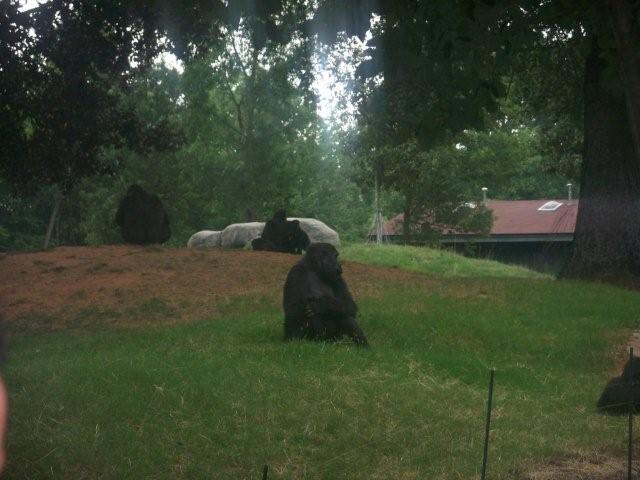In this outdoor zoo scene, three gorillas are situated on a grassy area with interspersed patches of brown dirt. Dominating the background is a large tree to the right, partially obscuring a small house-like structure with reddish roofing material and a couple of chimneys or vents. A thin fence with supports runs parallel to the back. 

The central focus is on a black gorilla in the middle of the image, seated with its arms crossed, gazing towards the left. In the background, slightly towards the upper left, another gorilla is walking away, its back turned to the camera. Additionally, near the lower right corner, a third gorilla is either lying or sitting with crossed legs next to an object resembling white plastic. The scene is framed by dark and lighter green trees, with a glint of blue sky peeking through, bathing the area in daylight.